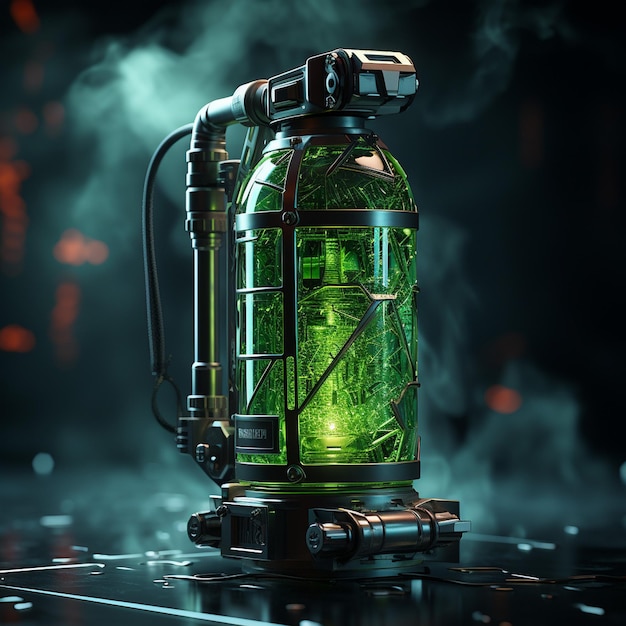A dramatic scene unfolds against a stark black background, tinged with wisps of gray smokiness that add an ominous atmosphere. The floor is laid with black tiles, and scattered across it are small gray drops or dots, contributing to the eerie setting. In the distance, faint red lights pierce the darkness, hinting at unknown machines or elements beyond view. Dominating the center of the image is a large, green glass canister encased in black plastic. At its base is a plastic roller, suggesting mobility or functionality within a larger mechanism. Extending upward from the canister are tubes that culminate in a sprayer, likely indicating the canister's purpose as part of a spraying or dispersal system. The detailed composition and varied textures of the elements draw the viewer into this mysterious and industrial tableau.